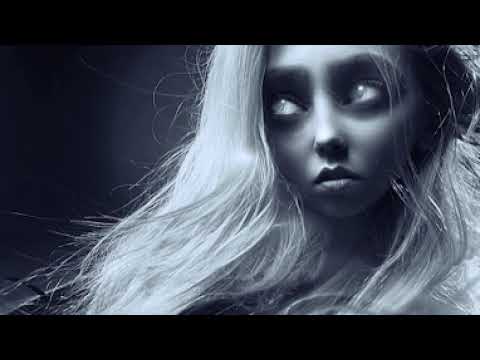This image appears to be AI-generated, focusing on a young woman depicted from the neck up with a cold blue-gray hue that lends the image a surreal, almost otherworldly quality. She is set against a background that transitions from black to a darker gray, framed by a black border at both the top and bottom. Her platinum blonde or possibly white hair cascades down, giving her an ethereal look. The woman gazes to her left with large, luminous eyes that lack detailed pupils, rendering them almost cataract-like, contributing to an uncanny, potentially blind appearance. Her facial features are sharply defined and angular, with an almost exaggeratedly realistic portrayal that borders on the alien-esque. Dark shadows around her eyes, deepened by the cold tonal filter, enhance the dramatic effect of the image.